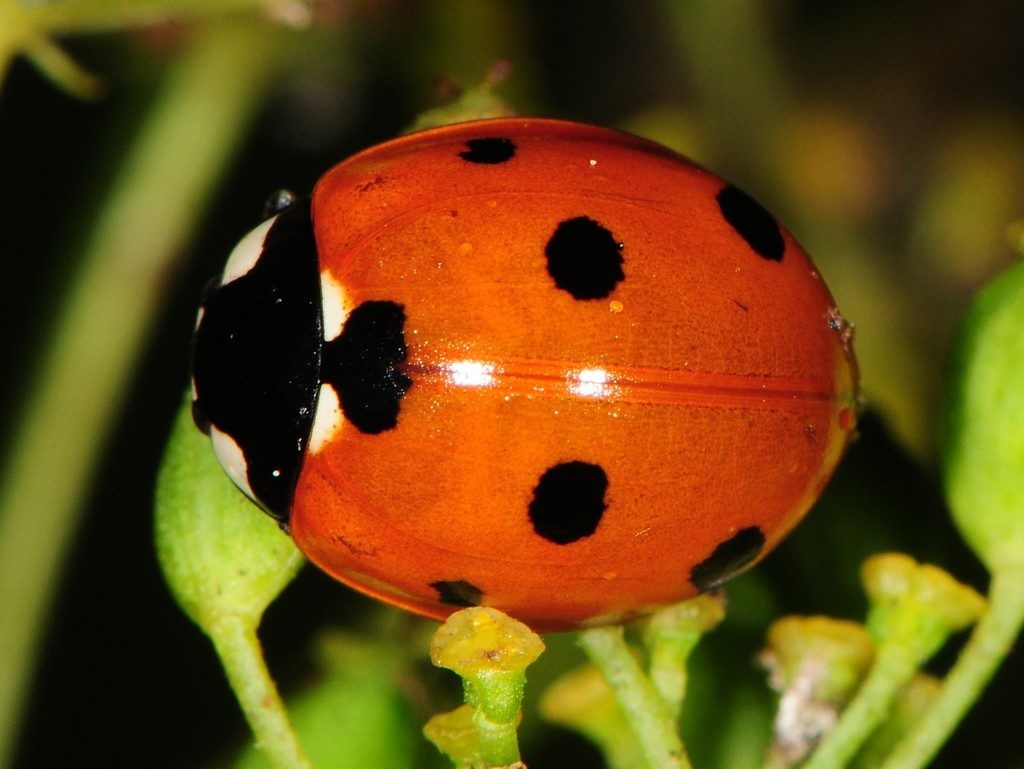This very detailed, high-resolution close-up photo captures a ladybug perched on a green leaf amidst blurred plant surroundings. The ladybug is oriented sideways, allowing a clear view of its oval-shaped back. The shell, while distinctly red, exhibits a faded, almost burnt, brownish-orange hue and features a symmetric pattern of black spots—three near the top, one in the center, and three towards the bottom—totaling seven spots. A faint midline runs down the middle, accentuated by the camera flash, creating two subtle white highlights. The ladybug's black head, adorned with white marks near the eyes, slightly peeks out from under the shell. The entire scene, with its dark, out-of-focus background and specks of water flicked across the ladybug and surrounding green foliage, highlights the insect's delicate beauty.